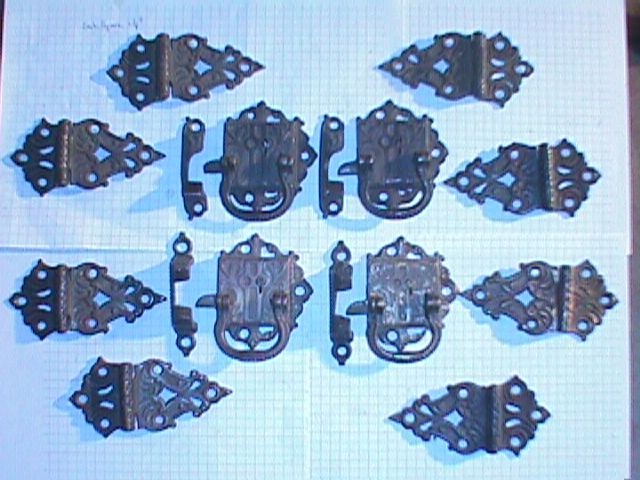The photograph features a carefully arranged collection of ornate antique hardware placed on a background of neatly aligned graph paper, typically used for plotting or drawing. The graph paper, characterized by its grid-like pattern of small squares, perfectly accentuates the detailed layout of the metal objects.

In the image, there are eight intricately designed wrought iron hinges, positioned in pairs. These black hinges, evocative of those you might find on a grand antique chest or a large jewelry box, contribute to the symmetrical arrangement. Centered among the hinges are several elaborately styled drawer handles resembling traditional door knockers. Additionally, the image includes front locking mechanisms and swinging handles that would lift open the lid of a piece of furniture. A small flat lock designed to accommodate a key is also visible.

The entire assortment appears to be part of an old, possibly antique set of drawers or a similar furniture piece. The hardware items, with their tarnished appearance, suggest they are aged and might be in the process of being cleaned or restored. The meticulous placement on the graph paper highlights each piece's ornate craftsmanship and fleeting historical charm.